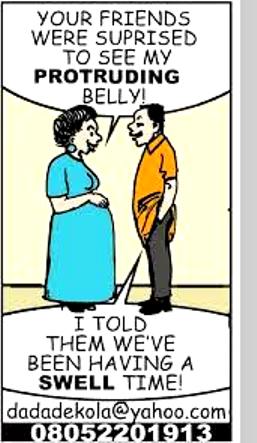This detailed comic strip features a woman with curly black hair wearing a blue dress, adorned with large circular earrings the same color as her dress. She appears pregnant and is speaking to a man dressed in a collared orange shirt, black pants, and black shoes, who has a slight beer gut. The top panel shows the woman saying, "Your friends were surprised to see my protruding belly." The man responds in the next panel, "I told them we've been having a *swell* time," with "swell" emphasized in boldface letters. At the bottom of the comic, on a black background with white text, is the email address "dadadekola@yahoo.com" and the number "08052201913." The background of the comic is a plain tan color.